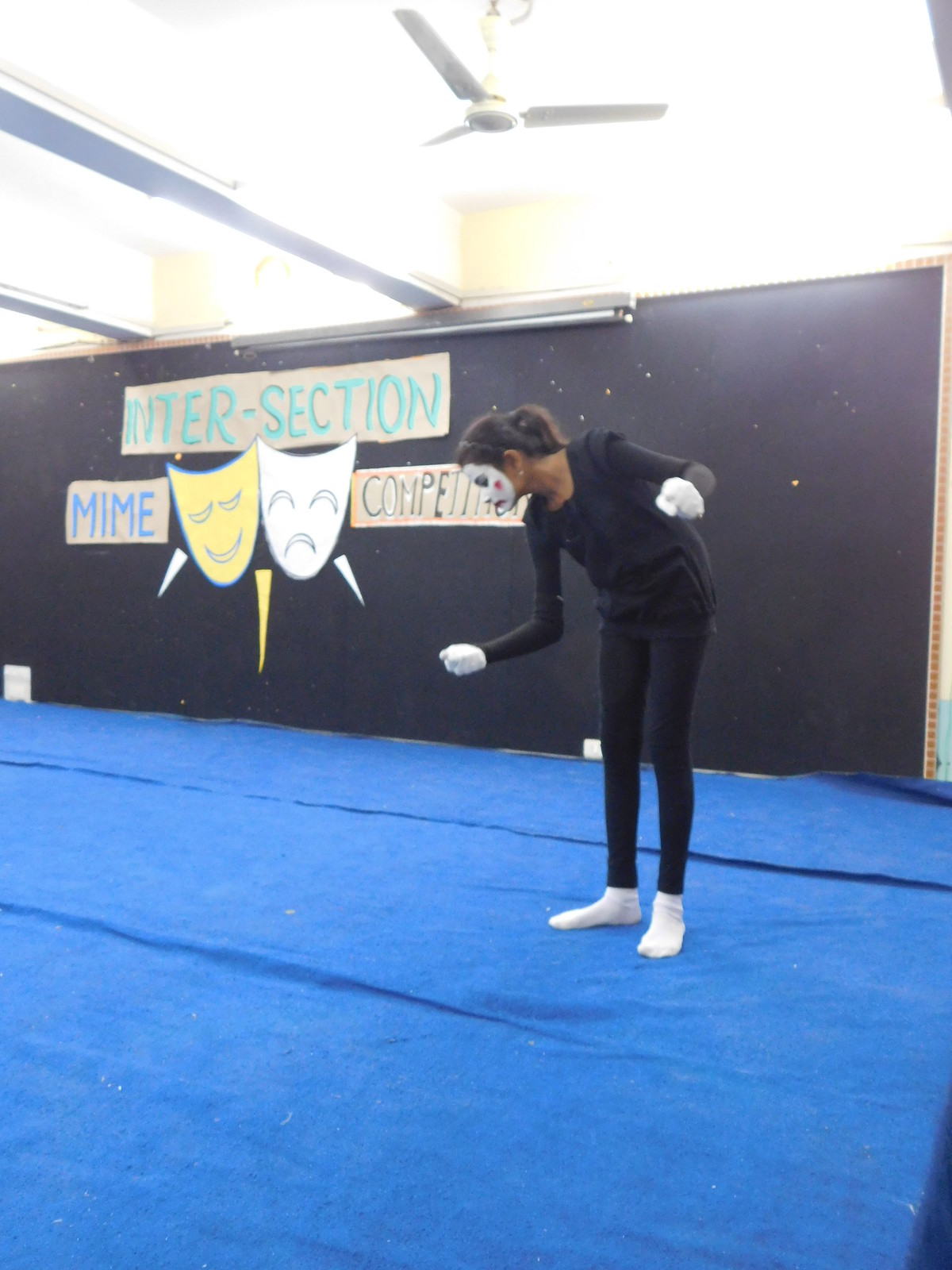In the image, a woman is participating in a mime competition. She is dressed in a traditional mime costume, consisting of a black long-sleeve shirt, black tights, white socks, and white gloves. Her face is painted in white mime makeup, complete with rosy red cheeks, which might initially be mistaken for a mask. She has shoulder-length dark hair pulled back into a ponytail and is looking down during her performance. She stands on a blue mat or tarp that covers the floor, possibly within a gymnasium. In the background, a large sign on the wall reads "INTERSECTION MIME COMPETITION" in blue and black lettering, accompanied by two images of mime masks—one yellow and smiling, the other white and frowning. The overall setting reinforces the context of the mime competition that the woman is actively participating in.